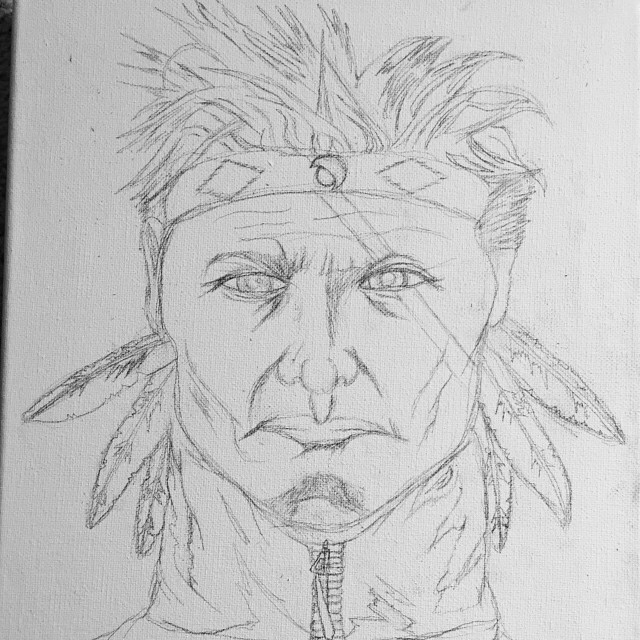This highly detailed pencil outline drawing captures the intense, direct gaze of a Native American man. His face, portrayed with striking realism, reflects a grim expression that adds depth to his character. He wears a headband adorned with intricate patterns, including a central crescent moon flanked by two diamond shapes. His unkempt hair protrudes from the top of his head, with feathers meticulously tucked into his locks, extending out at the sides. His thick neck is accentuated by a decorative piece running down its center, and hints of chin hair further enhance the lifelike quality of the drawing. The overall composition draws attention to the intricate details, emphasizing the artist's commitment to realism.